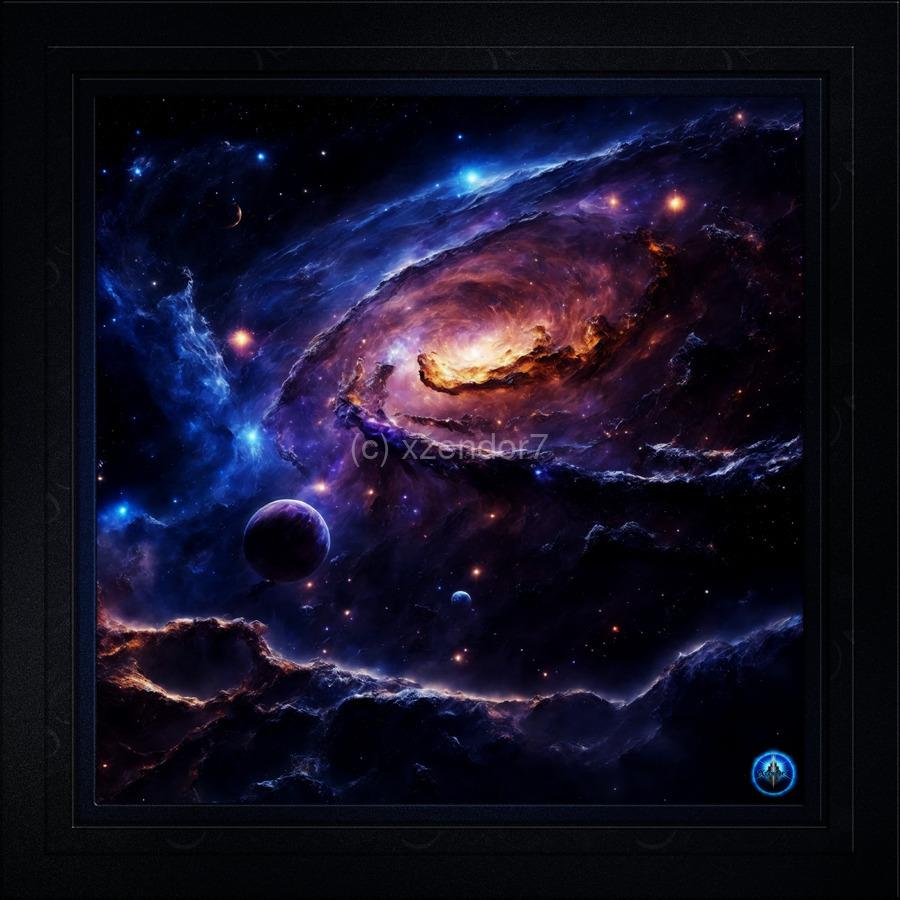This is a square AI concept artwork titled "Artreus Nebula" by Zendor7. The digital art features a stunning science fiction portrayal of a galaxy with a detailed spiral pattern, including its spiral arms set against a black sky. The center of the image is illuminated with blue swirls, and an array of dust clouds, stars, and celestial bodies in various colors. On the left side, a formation resembling a dragon's head with horns can be seen, adding an imaginative touch to the nebula's structure. The scene also includes the surface of what appears to be a moonscape or Mars scape at the bottom, along with multiple planets and stars. The primary light sources are yellow-orange, especially at the galaxy's core, contrasted by a blue star at the top of the frame and others on the left side. The image contains a watermark with "copyright XZENDOR7" at the center, and a mostly blue circular logo at the bottom right, further emphasizing its unique artistic quality.